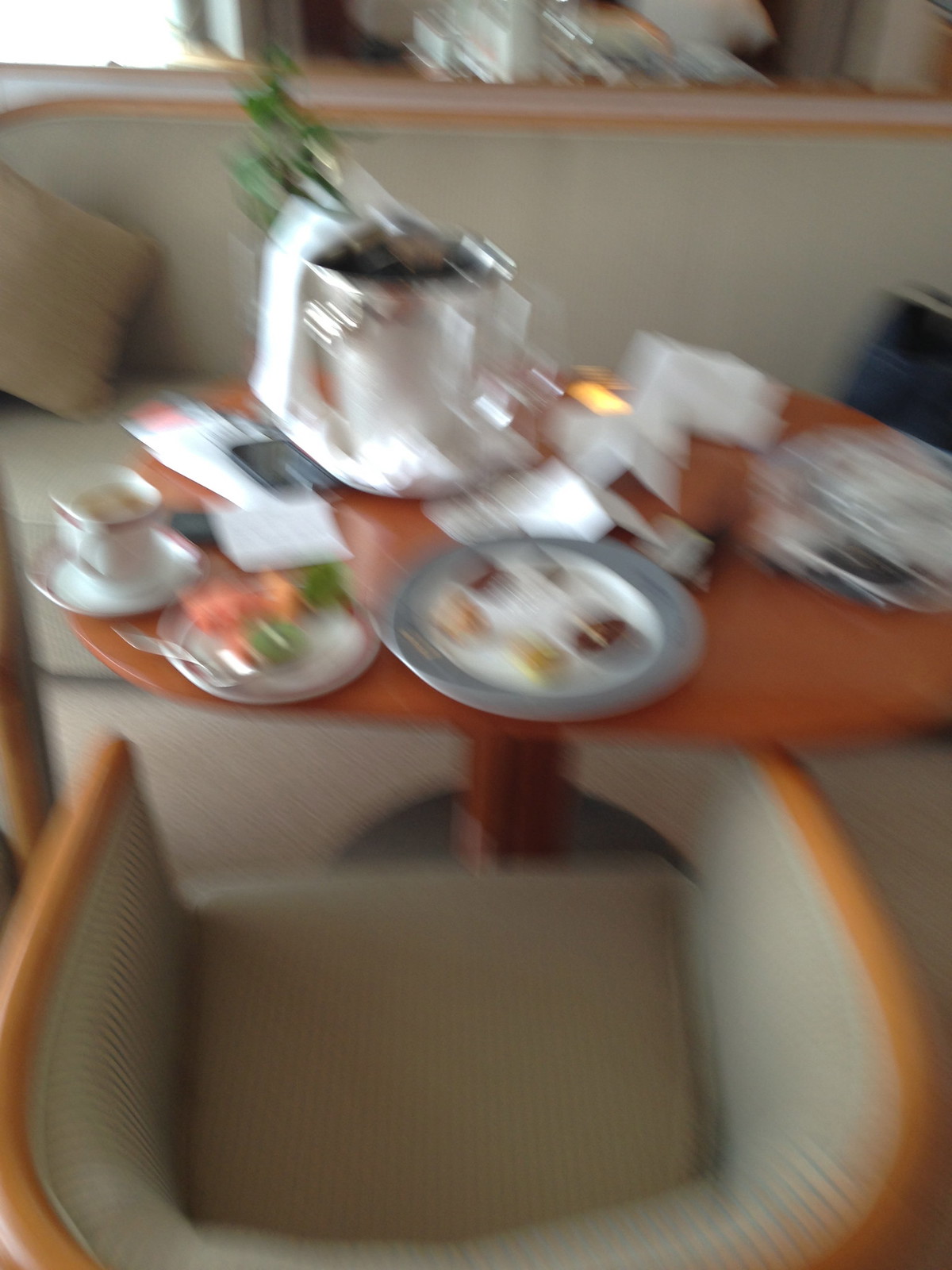A blurry photograph captures a meal setup inside what appears to be a hotel room, rather than a dining area. In the background, a beige couch with a wooden frame and a pillow is visible, accompanied by a matching chair with wooden armrests. The room's decor includes a wood table, which is the focal point of the image and is set for a meal, possibly breakfast. The table holds a plate of eggs on the left, an orangish dish beside it, and a small cup of coffee on a saucer. Scattered papers are visible near a large silver pot with greens sticking out of it, and a white cloth lies nearby. To the right, more papers are seen along with a plate and a bluish item resting on the couch. The table stands on a black base, which contrasts with the beige carpet underneath.